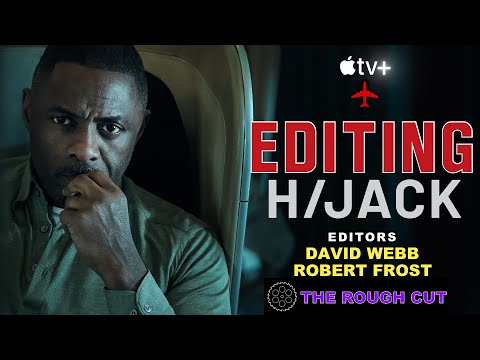This promotional image for the Apple TV Plus show "Hijack" features a prominent African-American man, seemingly around the age of 40 to 50, seated in an airplane. He appears deeply focused, with one arm raised near his chin. The black background accentuates the details in the scene. On the left, the man is dressed in a white, buttoned shirt, possibly resembling a jersey with three buttons at the top. He is visibly frowning as he gazes intently, likely at an in-flight screen. 

On the top right in white font, there’s the recognizable Apple TV Plus logo, consisting of the iconic bitten apple followed by "TV+" in white print. Directly beneath this logo, there is a small, red airplane graphic. Below this, the word "Editing" is prominently displayed in large, bold red letters with a white outline, followed by the show's title "Hijack" in standard white font. Further down, in yellow font, the text lists the editors, David Webb and Robert Frost. The caption culminates with the phrase "The Rough Cut," written in large, purple letters with a white outline.

Together, these elements create a detailed advertisement highlighting the show's editing team for "Hijack" on Apple TV Plus.